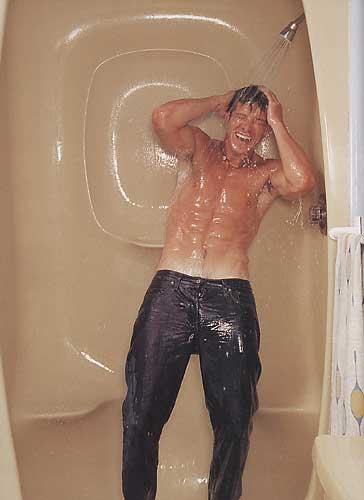This photograph captures a man standing under a running shower inside a beige-colored shower stall. The shower wall behind him features a distinctive spiral circle and a rounded rectangle pattern towards the lower section. Positioned to his left is a white shower curtain, while the lower right corner reveals the edge of a sink top. To the right side of the frame, additional details include a towel rack with a hanging towel and the toilet tank lid.

The man is notable for his unusual attire in this setting: he is shirtless but wearing long, dark pants that are either black or dark blue. The pants are soaking wet, along with his face and chest. The shower spray, directed from above his head, streams down, drenching him completely. The man's hands are in his hair, as though he is washing it, and his eyes are shut. His face is lit up with a broad open-mouth smile or laugh, likely reflecting the humor he finds in standing in the shower fully clothed.